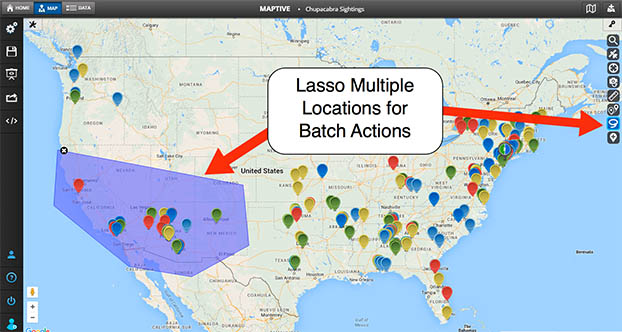The image is a detailed map of the United States, partially extending to the bottom of Canada and portions of Mexico, captured from a computer screen, likely from a webpage or an app. Dominating the map are various colored pinpoints—yellow, blue, red, and green—which are mostly concentrated in the central, northeastern, and somewhat southwestern regions of the U.S. At the top of the screen, a black navigation bar with icons like the home button and map button can be seen, while a black side panel on the left features other functional buttons including a save button.

In the center of the map is a prominent white text box with rounded corners, containing the phrase "Lasso Multiple Locations for Batch Actions" in black lettering. Two red arrows extend from this text box, one pointing towards the lower west coast and another towards the upper east coast. Additionally, a grey, transparent rhomboid shape overlays portions of Southern California, extending down to Baja, Mexico, and into Texas, allowing the underlying map details and pinpoints to remain visible. The application appears to be from a program called "Maptive," as indicated by the title at the very top of the image.